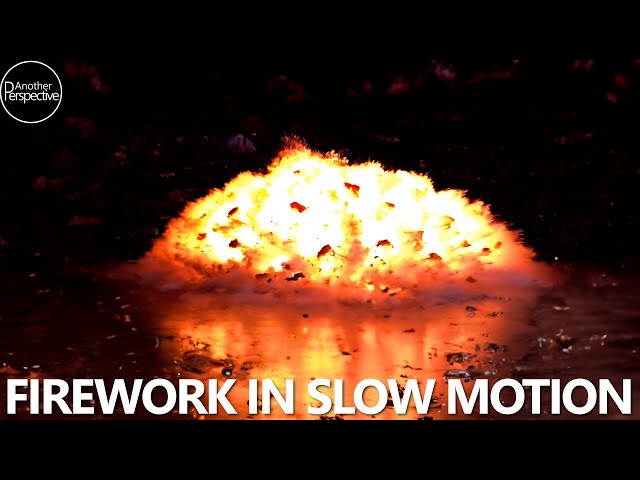The photograph, possibly an advertisement, features a striking scene with a black background, punctuated by several small points of orange light. At the center of the image, a blazing firework explosion dominates, showcasing a bright yellow core that transitions to darker hues of orange as it radiates outward. This explosion is captured in slow motion, with debris and firework residue visibly blowing outward from the center. The ground in front of the flames appears to be wet or shiny, mirroring the explosion, albeit less intensely. The reflective surface enhances the dramatic effect of the firework. In large white lettering across the bottom, the words "Firework in Slow Motion" are boldly displayed, while the phrase "Another Perspective" is inscribed in white within a circle located in the top left corner.